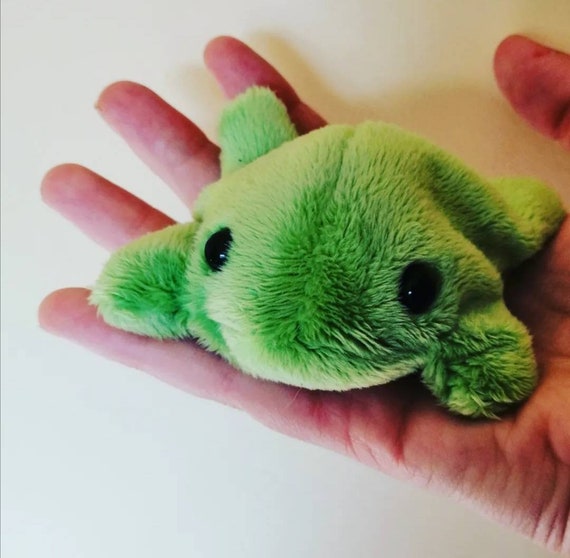The image features a close-up of a small, green stuffed animal frog cradled in a lightly colored, somewhat wrinkled hand. The hand enters the frame from the bottom right corner, with the palm and four fingers visible, extending to support the frog, though the thumb remains slightly detached, coming from the upper right corner. The background is a smooth, white wall, and a light source creates subtle shadows, accentuating the furry texture of the frog. This plush frog is approximately palm-sized, with medium green fur, and has four legs splayed out to the sides. The frog's two black beaded eyes gaze directly at the camera, giving it a friendly appearance. Additionally, it has a light green to white underbelly and a faint seam running down its spine. The overall scene captures the endearing nature of the frog and the gentle manner in which it is held.